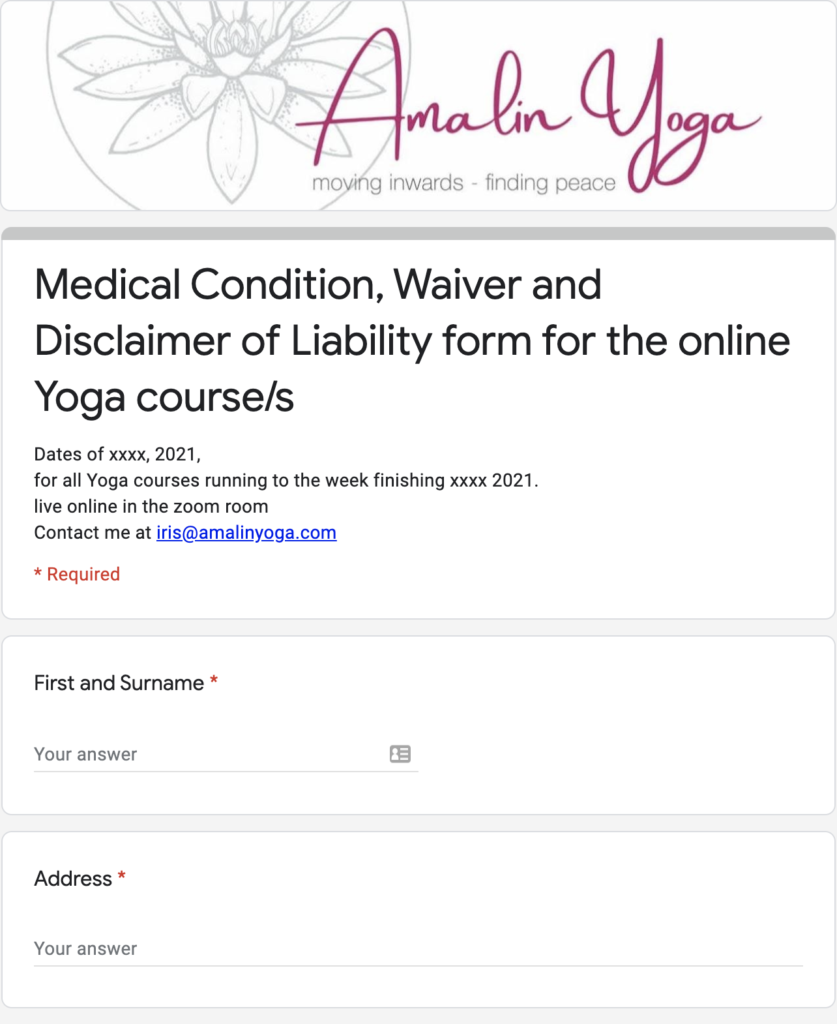Under the heading "Websites," the top section features a light gray background with a central circle containing a lotus flower design, drawn in gray on white. Beneath the circle, in prominent purple letters, it reads "Amalin Yoga," followed by the tagline "Moving Inwards, Finding Peace." Below this is a formal document titled "Medical Condition Waiver and Disclaimer of Liability Form for the Online Yoga Course," with several dates indicated as "Blank 2021" through to the end of a certain week in "4X's 2021." This document is intended for participants of live online yoga courses conducted via Zoom.

For further inquiries, users are instructed to contact the organizer at iris@amalinyoga.com, with the email address highlighted for easy access. The form includes a required field for the participant's first and surname, denoted by a red asterisk. There is also a field for the address marked with an asterisk indicating it is mandatory, alongside a line provided for filling in the response. The form is presented in a white book format with black writing, with the required fields and indicators prominently marked in red.